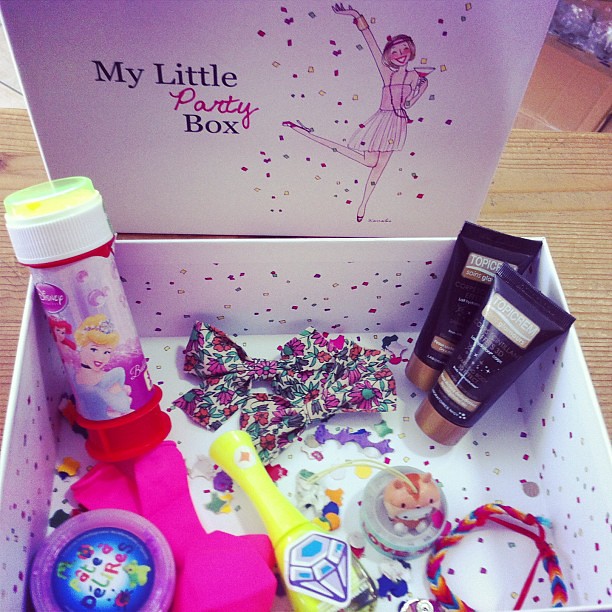The image depicts a festive scene featuring "My Little Party Box," set on a wooden table. The box lid, visible in the background, showcases a colorful drawing of a woman in a sleeveless pink dress, with her leg kicked back and hand raised amid confetti as if celebrating. The illustration, done in a colored pencil style, adds a whimsical touch to the presentation.

Inside the box, colorful confetti lines the bottom, enhancing the festive atmosphere. Prominently displayed is an orange bottle with a white twist cap, adorned with a sticker of Disney princesses like Cinderella and the Little Mermaid. Accompanying this are two floral bows, each designed with pink and white patterns. There are two brown and gold tubes labeled "Topicrem," assumed to be beauty products. Additional playful items such as a tiny plastic container of modeling gel, a couple of pink rubber balloons, a bubble solution container, and a multicolored bracelet complete the assortment of knick-knacks found inside. The varied contents suggest a mix of beauty supplies and toys, possibly targeting a wide age range and creating an eclectic, party-themed collection.